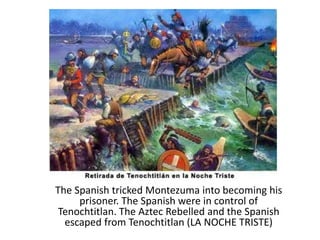The small, square informational graphic features a vivid painting depicting a historical battle. At the top of the graphic is the painting titled "Retirada de Tenochtitlan en la Noche Triste," which translates to "Retreat from Tenochtitlan on the Sad Night." Below the painting, in small black letters, this title is repeated. The typographic details narrate that the Spanish tricked Montezuma into becoming their prisoner, gaining control of Tenochtitlan. However, the Aztecs soon rebelled, forcing the Spanish to escape in an event referred to as "La Noche Triste."

The painting is dynamic and detailed, filled with the chaos of battle. It illustrates Spanish soldiers in small wooden boats, armed with bows and arrows and shields, while Aztec warriors confront them from both water and land. The scene shows soldiers and horses struggling in the tumult, some appearing to leap from boats to land while others are in the river or crawling up the banks, possibly indicating the Aztecs' fierce retaliation. The vivid colors—blues, greens, golds, and browns—highlight the intensity and drama of this historical confrontation.